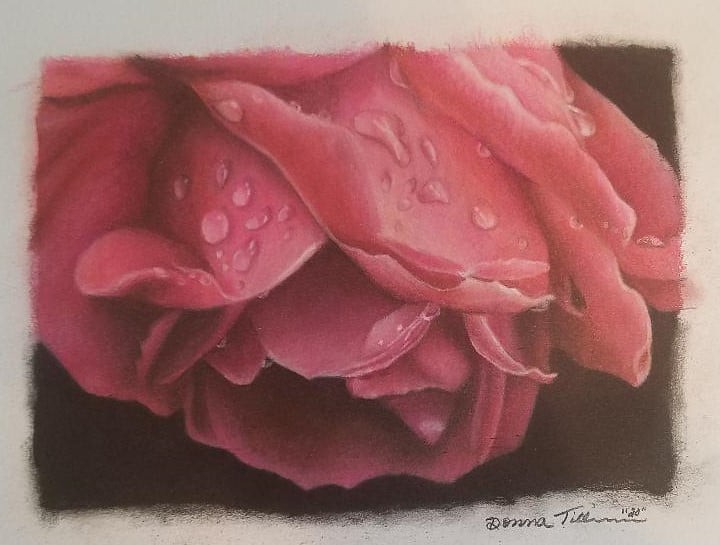This painting features a collection of pink flower petals, prominently displayed and forming a dense cluster that occupies the majority of the composition. The petals are delicately painted to illustrate varying shades of pink, with the top petals adorned with realistic water droplets, adding a touch of freshness and life to the artwork. The background sets a striking contrast, being a deep, dark brown that enhances the vividness of the petals. Encasing the painting is a light gray frame, which subtly complements the darker tones within. In the bottom right corner, a black cursive autograph is visible, marked with the number "20" in quotation marks. This detailed interplay of colors, textures, and subtle elements creates a captivating floral representation.